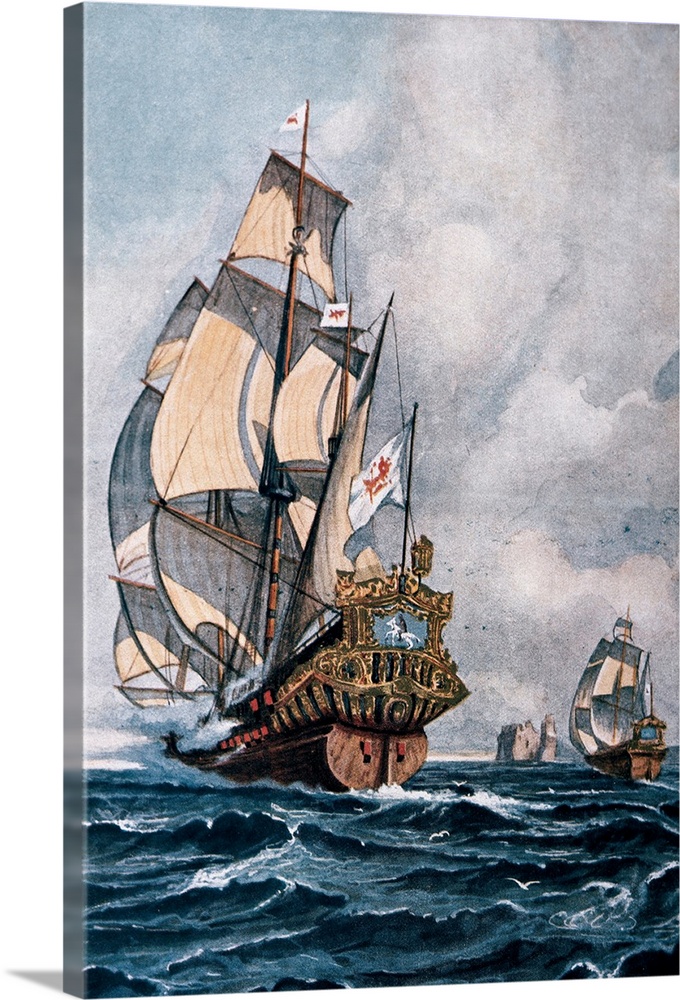A meticulously detailed painting depicts a dramatic ocean scene with two wooden sailboats navigating through tumultuous, dark blue waves under a cloudy sky. The focal point is a large, brown-hulled ship with distinctive white sails and a white flag adorned with a simplistic red dragon head marked with needles along its nose. The ship is gold-encrusted at the stern, showcasing a blue portrait of a man in dark blue attire riding a white horse. To the right of the main ship, a smaller but similarly designed boat sails nearby. In the distant background, an island is topped with what appears to be a castle or possibly large rocks, adding a sense of depth and mystery to the composition. The overall tone of the painting is dark and moody, capturing the peril and grandeur of seafaring life.